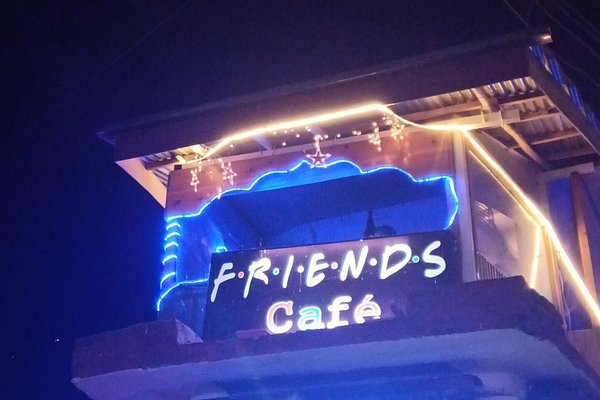In this nighttime image, a sign for "Friends Cafe" is prominently displayed on the second floor of a small building, outlined with neon lighting. The sign explicitly uses the iconic style of the TV show "Friends," with each letter of "F.R.I.E.N.D.S" separated by a dot and illuminated in white neon, while the word "Cafe" includes accents of blue neon in the letter "A." The scene is dark with minimal surrounding light, except for the sign and some ambient lighting. Blue neon rope lights wrap around one of the supporting posts of the structure, which resembles a wooden tower or pavilion with a corrugated metal roof. Additionally, white rope lights adorn the roof, and a few small illuminated stars hang beneath it, adding a festive touch. Power lines are visible on one side, further grounding the scene in its slightly rustic setting.